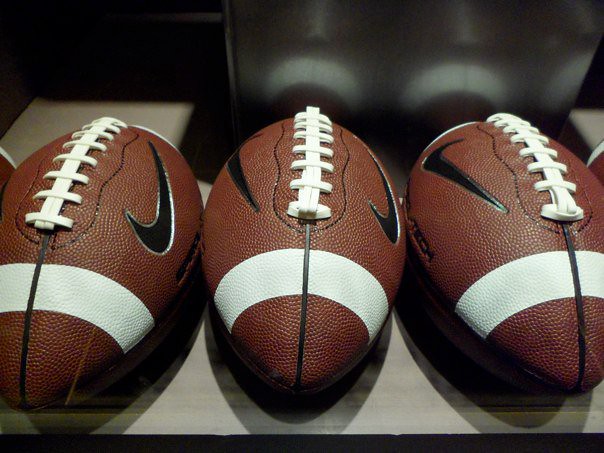The photograph is a professional, slightly underexposed color image depicting three brand new, large Nike-branded rugby balls meticulously placed side by side on a polished wooden shelf. The balls are arranged with the central ball pointing directly at the viewer, flanked by the other two balls turned slightly outward in a diagonal formation. Each rugby ball, made by Nike, features a terracotta color with distinctive white stripes encircling both ends and thick white laces running up the middle. The Nike logos, black with silver or white highlighting from the light source, are prominently displayed on the sides of each ball. The background features a blurred black shiny surface, enhancing the composition with a subtle reflection of the balls' white details. The whole setup conveys an immaculate, glossy appearance suggestive of a high-end advertisement for a magazine or a website.